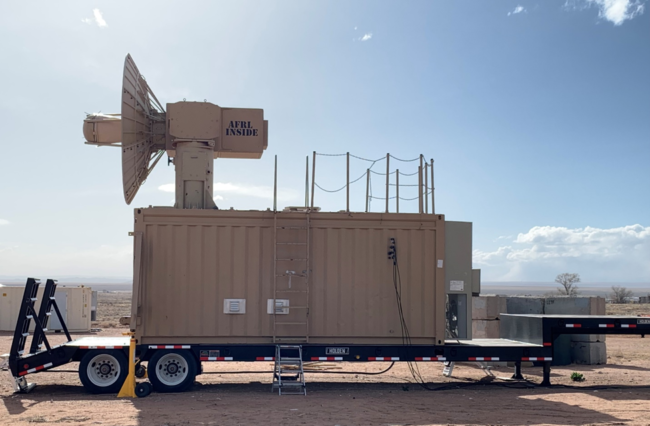The photograph captures a large machinery setup situated in an open, sandy field with minimal plant life and a few distant trees. The central feature is a flatbed trailer designed to be pulled by an 18-wheeler truck, complete with black wheels. Atop this flatbed sits a beige-colored metal shipping container with ridged sides. Affixed to the shipping container is a small step ladder leading to an attached metal ladder with a chain and metal stake railing.

Positioned at the far end on top of the container is a sizable satellite dish apparatus, also painted in the same light khaki color as the container. The dish is oriented to the left of the image and prominently displays the letters "AFRL" in bold, black font. The scene is set under a partly cloudy sky, with light blue hues and scattered white clouds, adding to the expansive desert atmosphere.